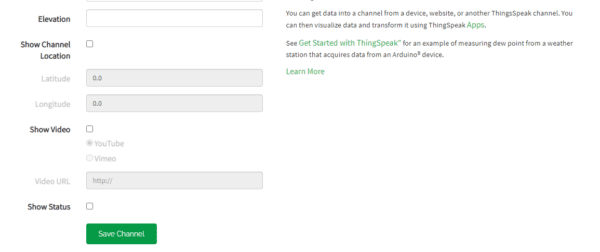The image depicts a web page with a predominantly white background, displaying a mixture of black and green text. On the left side, there is bold text that reads "Elevation," with an adjacent empty rectangular box. Beneath that, another bolded heading, "Show Channel Location," appears with an empty square box next to it. The sections for "Latitude" and "Longitude" are highlighted, each accompanied by a box containing the value "0.0".

Further down, "Show Video" is bolded, with the corresponding square rendered as shaded. The options "YouTube" and "Vimeo" follow, where "YouTube" is both checked and shaded. Below this, there is a section labeled "Video URL," also shaded, with a box containing the text "HTTPS."

Toward the bottom of the image, the bold text "Show Status" is displayed with an empty square box alongside it. The web page prominently features a green button labeled "Save Channel" near the lower right area.